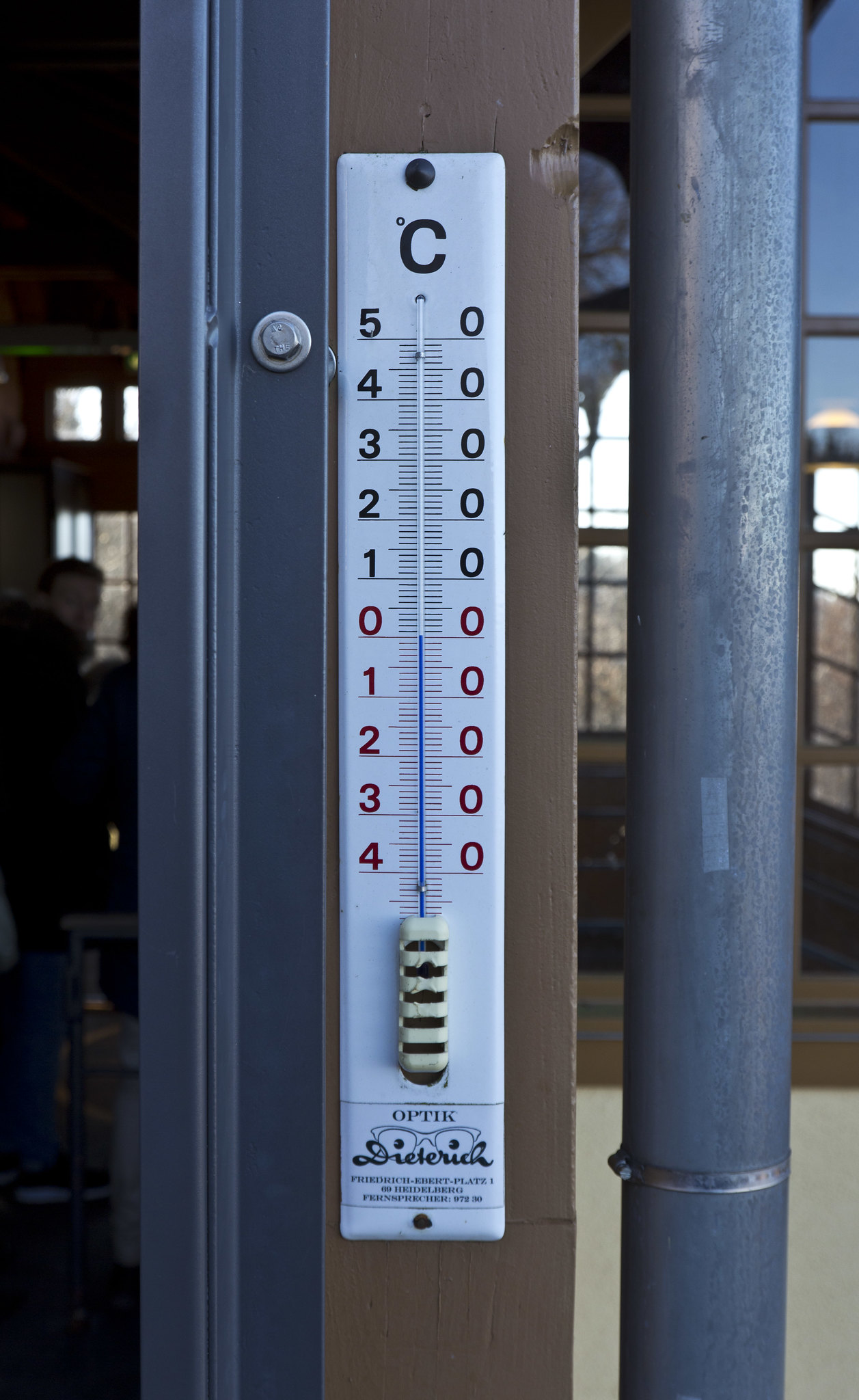This photograph features a centigrade thermometer prominently mounted on a vertical post, situated centrally in the image. The thermometer displays a dual scale with temperatures marked in both black and red numerals. The left side of the scale runs from 5 down to 1 in black, then transitions to red for 0, and continues downward to 4. On the right side, the scale prominently features ten zeroes in succession, equally spaced. At the top, the thermometer is marked with a "°C" symbol, indicating its measurement in Celsius.

The thermometer has two mounting holes, one at the top and another at the bottom. The bulb at the base of the thermometer is striped in yellow and black. Beneath the bulb, there is a logo for "Optik," featuring the text "O-P-T-I-K" alongside a pair of eyeglasses with black dot eyes. Below this logo, there may be the word "Dietrich" and additional, unreadable lettering.

Adjacent to the thermometer, on its right, is a gray metal pipe. On the left side, a metal bracket with a bolt is visible, positioned near the “5” and “4” marks on the thermometer. This bracket spans horizontally across the width of the photograph and matches the gray color of the pipe.

The background hints at an outdoor setting, possibly near a ski lodge or restaurant, with patches of snow visible in the upper right section of the image and a glimpse of blue sky overhead.